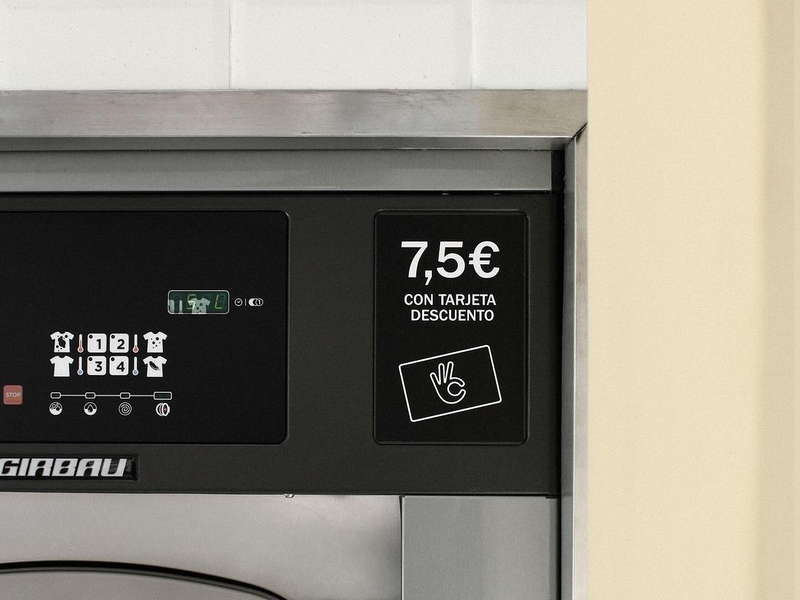The image depicts the upper right corner of a silver washing machine, likely located in a laundromat. The machine features a range of symbols and texts, predominantly in Spanish. A white wall frames the picture, suggesting a tiled backdrop. On the left side, there's a display panel with icons of t-shirts alongside numbers 1, 2, 3, and 4, each paired with a small thermometer, likely indicating different washing settings or temperatures. Below this, a progress bar is visible, adorned with various smaller symbols. The central area contains a black section with a digital display showing the number "0". The brand name "GIRBAU" is present, signaling the machine's maker. On the right side, text in Spanish reads "con tarjeta descuento," which translates to "with discount card," and it includes a "75¢" cost indication, marked with a currency symbol resembling a "C" with two lines through it. Additionally, a rectangle containing a hand making an "OK" gesture is seen, possibly illustrating a card insertion point or a user indication.